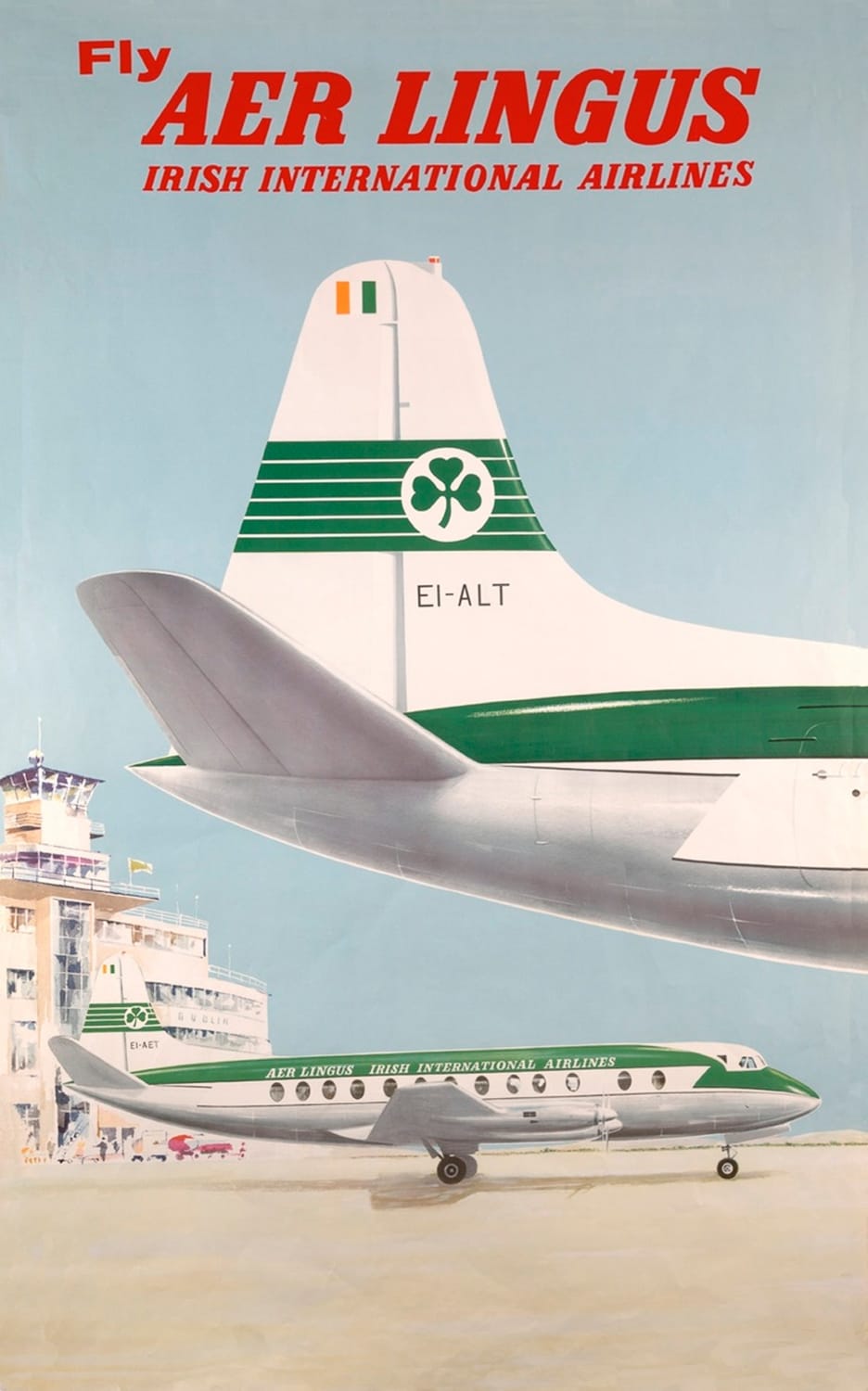The image appears to be an advertisement for Aer Lingus, the Irish International Airlines. Dominating the center of the image is the tail section of an airplane, depicted facing roughly the three o'clock position. This tail is primarily white, decorated with five horizontal green stripes. Prominently, a three-leaf clover, symbolizing Ireland, is featured on the vertical fin. Above this central airplane tail, red text reads, "Fly Aer Lingus, Irish International Airlines." In the background, there is a full airplane of the same design, occupying about 20% of the left to right section of the image and also oriented towards three o'clock. Additionally, the backdrop includes a building, contributing to the overall setting of an airport advertising scene.